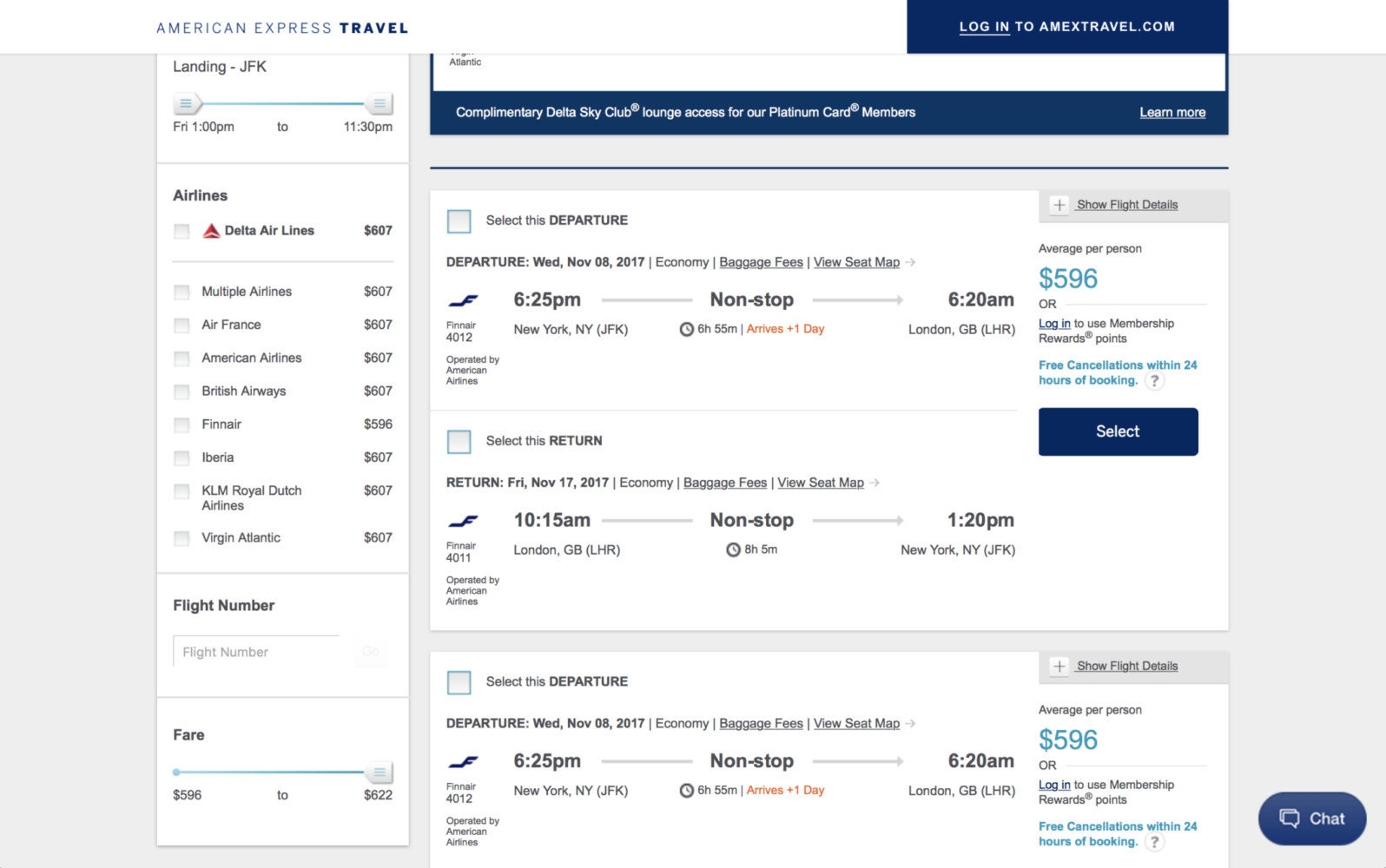The image is a screenshot of the American Express Travel website, showcasing its user interface and functionalities. At the top, the site prominently displays the American Express Travel logo with a prompt to log in to amextravel.com. On the bottom right corner, there is a chat button for customer support. 

Central to the image is the flight search results, highlighting various available options. In particular, there's a Finnair flight 4012, operated by American Airlines, departing from New York JFK at 6:25 PM, and arriving non-stop in London, Great Britain at 6:20 AM the following day. Another flight listed is a return trip on Friday, November 17, 2017, in Economy class. This flight departs London at 10:15 AM for a non-stop trip back to New York JFK, landing at 1:20 PM.

Additionally, there is another Finnair flight 4012, also operated by American Airlines, departing on Wednesday, November 8, 2017, from New York JFK at 6:25 PM, and arriving in London at 6:20 AM. The average price per person for these flights is displayed as $596.

On the left side of the screenshot, there is a sidebar with various filter options, allowing users to select airlines such as Delta Airlines, British Airways, American Airlines, Air France, Finnair, Iberia, KLM Royal Dutch Airlines, and Virgin Atlantic. Users can also search by flight number, filter by fare price range, and specify preferred landing times.